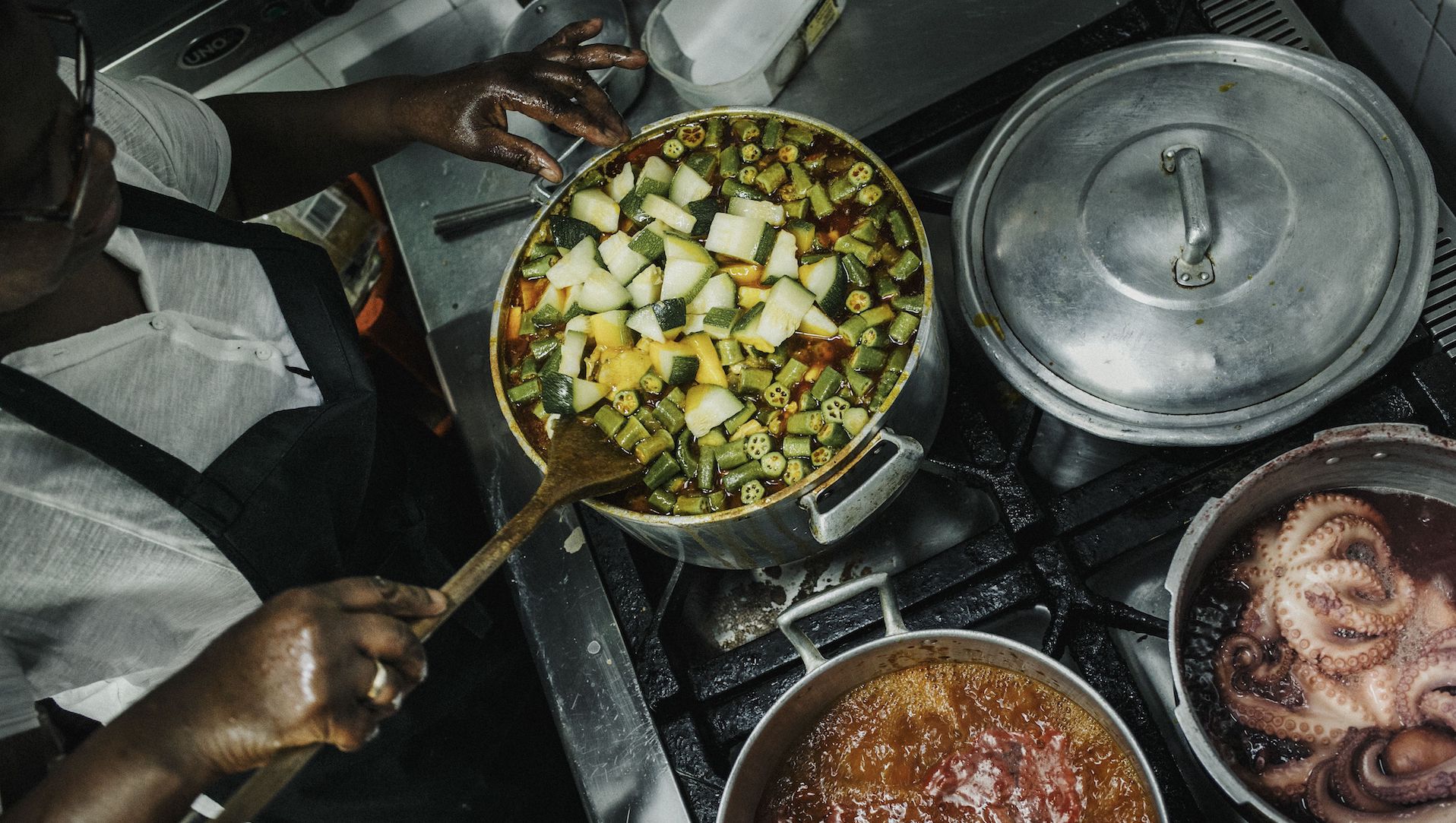This overhead photograph captures a bustling scene in an industrial kitchen where a black woman is actively cooking at a well-used, four-burner stove. She is wearing glasses, a white button-down shirt, and a black apron. Her right hand stirs a pot with a long wooden spoon, while her left hand steadies the rim. This pot, located on the top-left burner from the viewer's perspective, is brimming with various green vegetables, including okra, zucchini, and squash, immersed in a brown broth. In the top-right corner, a pot with a silver lid conceals its contents. The bottom right burner displays a pot with octopus submerged in a brown broth, tentacles visible as they curl upwards. On the bottom-left burner, a pot filled with a rich, reddish-brown liquid appears to have some sort of gravy or braising liquid. The stove bears the marks of extensive use, indicating a space that sees frequent and robust cooking activity.